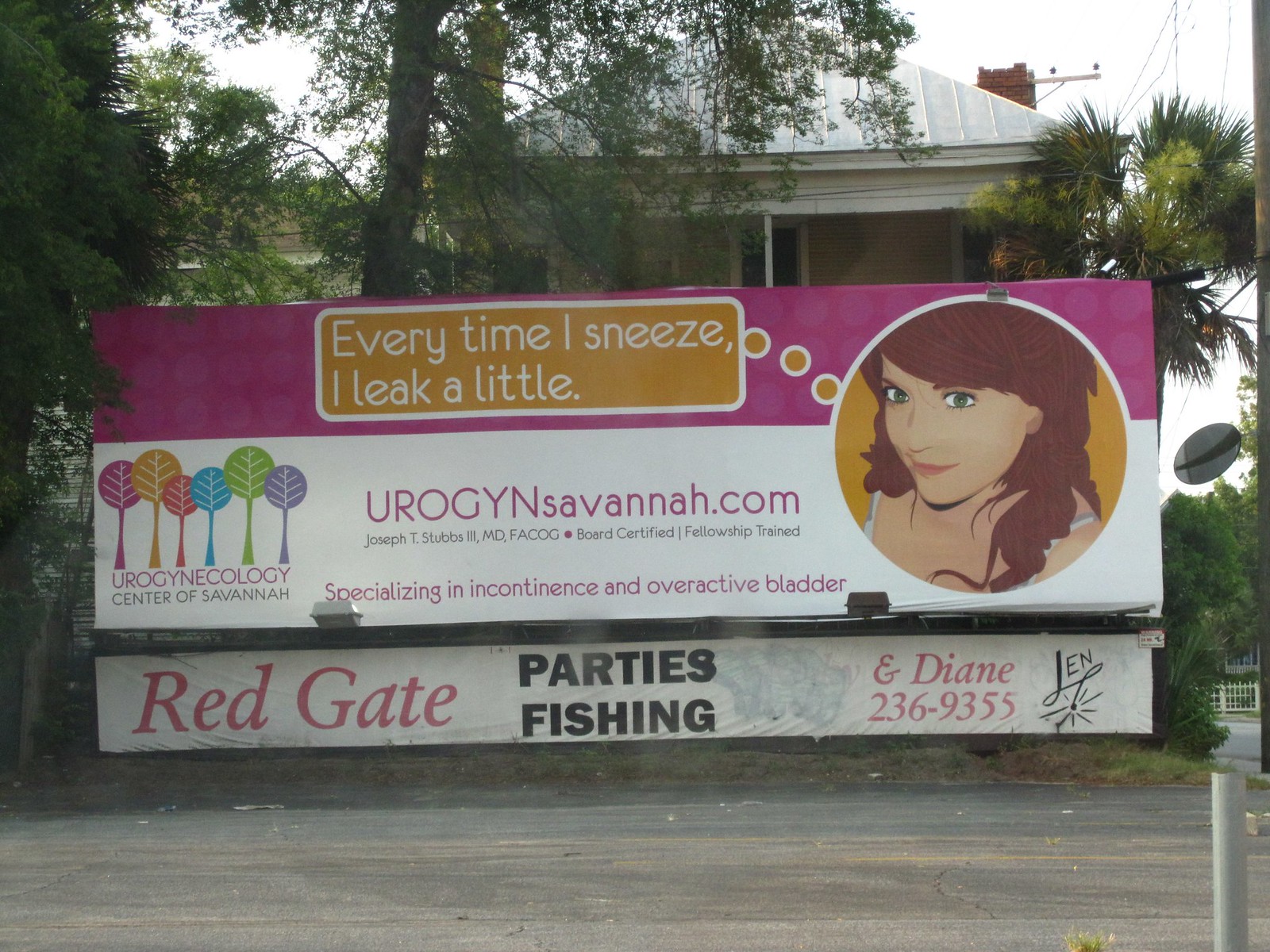This color landscape photograph captures two billboards positioned one above the other, seen from across a road. The photo is taken at the same height as the billboards, with a road visible at the bottom of the image, in front of a white house with a pitched roof and surrounded by a few trees. The top billboard, which is larger, is divided into a bright pink upper half and a white lower half. A circle within the billboard contains a cartoon image of a woman in her 20s or 30s, with brown hair, green eyes, and white skin. From the circle, a speech bubble in orange text reads, "Every time I sneeze, I leak a little." The sign advertises a urology medical practice with the website "urogyndsavannah.com" and mentions, "James T. Stubbs III, MD, FACOG, specializing in incontinence and overactive bladder." The bottom billboard, smaller in size, reads, "Red Gate Parties Fishing" and includes a phone number, "236-9355." There is a hint of graffiti on this smaller sign. In the background, hints of trees and the roofline of the house add context to the scene, while natural light highlights the vivid colors of the billboards.